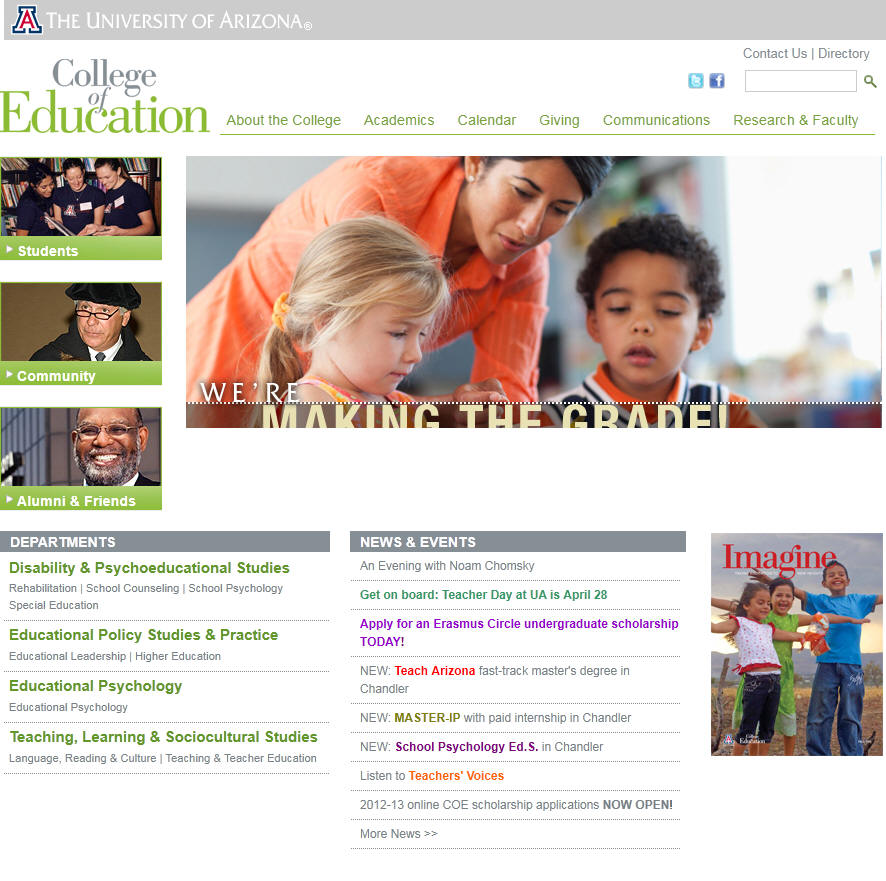At the top of the image, the bold block letter 'A' prominently features beside the name "University of Arizona" in blue, and "College of Education" in green. To the right, the menu options listed in green include: "About the College," "Academics," "Calendar," "Giving," "Communications," "Research," and "Faculty." Above this menu is a search bar with options to share on Facebook, contact the university, and access the directory.

Beneath "College of Education" is an image of students wearing black t-shirts, standing together in a library, and examining a book. Below this photograph is the word "Students." Adjacent to this is the image of a man wearing small black glasses and a black hat with the word "Community" underneath. Adjacent to "Community" is a smiling man with glasses and a gray and black beard, under the label "Alumni and Friends."

In the center of the image, a woman, presumably a teacher, is surrounded by two young children. They are looking down, possibly at a piece of paper or a book, with the caption "We're making the grade."

Finally, in the lower corner, the word "Imagine" is displayed in red text above an image of three children standing with their arms outstretched. The children include a boy in a blue shirt, a girl in a green dress, and another girl in a white and red top.